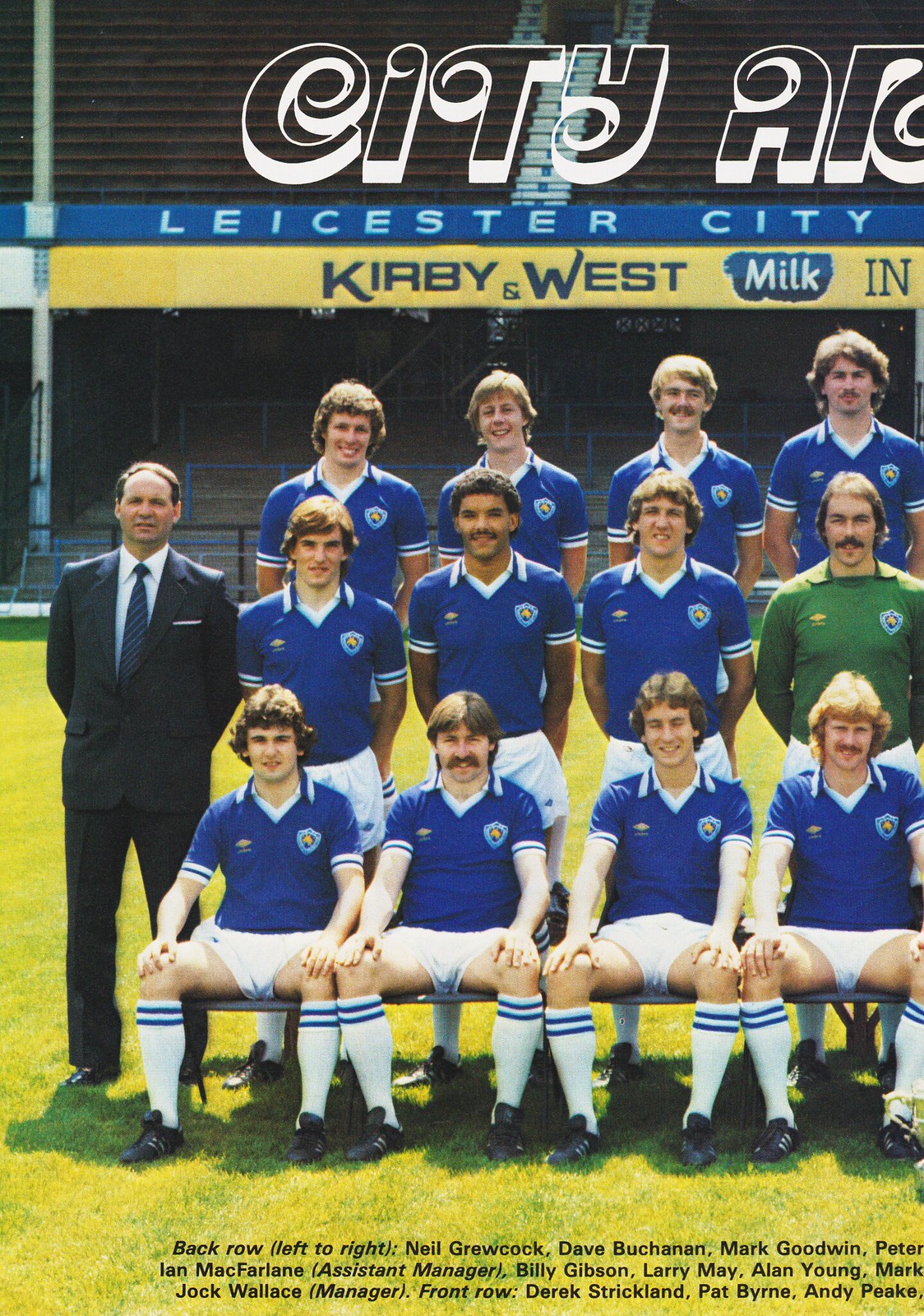In this team photo, the backdrop features a blue and yellow banner. The blue section at the top reads "Lancaster City," while the yellow section below includes partially visible text; "Caribbean West Milk Inn" is discernible before it's cut off. The team, dressed predominantly in blue shirts and white shorts, is arranged in three rows; the top two are standing, and the bottom row is seated on a bench. Notably, one man in the middle row on the far right is wearing a green shirt, and another on the far left, who is standing, is dressed in a suit. At the bottom of the image, black text provides names for some team members: 

Back Row (Left to Right):
- Neil Grukov
- Dave Buchanan
- Mark Goodwin
- Peter (cut off)
- Ian McFarlane (Assistant Manager)
- Billy Gibson
- Larry May
- Alan Young
- Mark (cut off)

Front Row:
- Jock Wallace (Manager)
- Derek Strickland
- Pat Byrne
- Andy Peake (cut off)

The rest of the names and text are not fully visible.